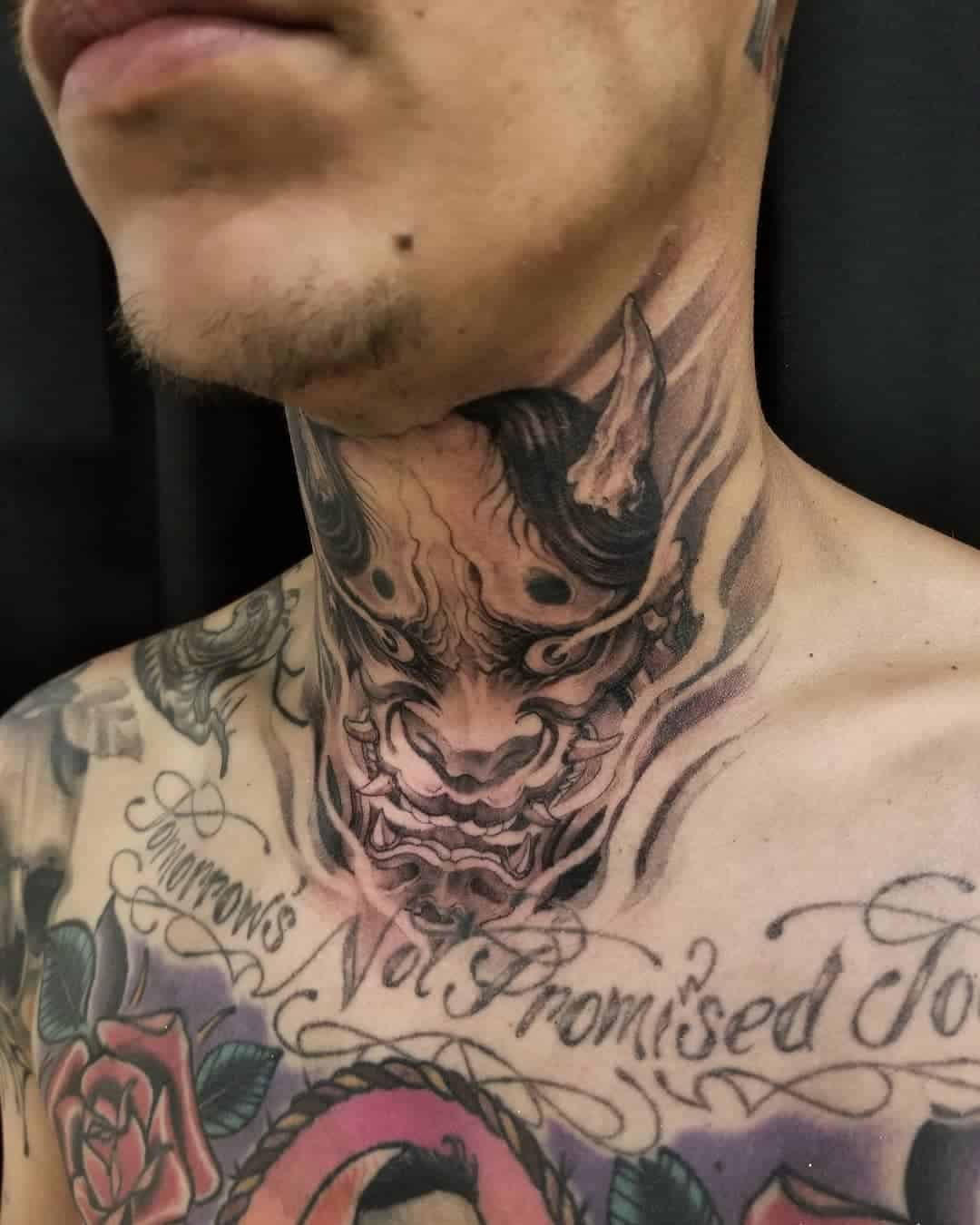This close-up, vertically aligned rectangular image captures the lower part of a man's face, from just above his lips to his chest, with his tan skin and a hint of dark brown scruff on his chin. Dominating his neck is a massive, intricate tattoo of a horrific creature with bulging eyes, sharp teeth, and devil horns. Smaller horns protrude from the sides of the creature's cheeks, and black hair flows around it. Below this foreboding figure, the words "Tomorrow's Not Promised" are inscribed in fancy black ink, though the right side of the text trails off and is cut off from view. This text and the design extend slightly over his shoulder.

On the left side of his chest, a vibrant red rose with green leaves is prominently displayed. Adjacent to this, partially visible, is a large O-shaped design with a rope border, transitioning into shades of pink, purple, and green. Centered on his chest, faintly discernible, is the beginning of a portrait, featuring what appears to be the head of a person with brown hair wearing a rimmed hat or hoodie. This tattoo composition creates a striking, eclectic array of imagery and colors, weaving a narrative of dark, whimsical artistry across his upper body.